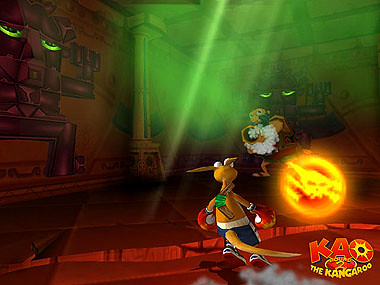In this animated or video game graphic, the scene features a cartoon kangaroo named K.A.O. from "Round 2: The Kangaroo." The kangaroo is dressed in blue boxing shorts and sneakers, with red boxing gloves on both hands, and is positioned with its back to the camera. In the background, a mysterious creature is sitting on a log that has a skull and crossbones marking, giving a sense of foreboding. The creature is holding something white in its hands, adding to the eerie atmosphere. The room is illuminated by an unsettling green light with vertical beams. On the left side of the image, the walls are decorated with various geometric patterns and highlighted green eyes, enhancing the eerie and suspenseful mood of the scene.